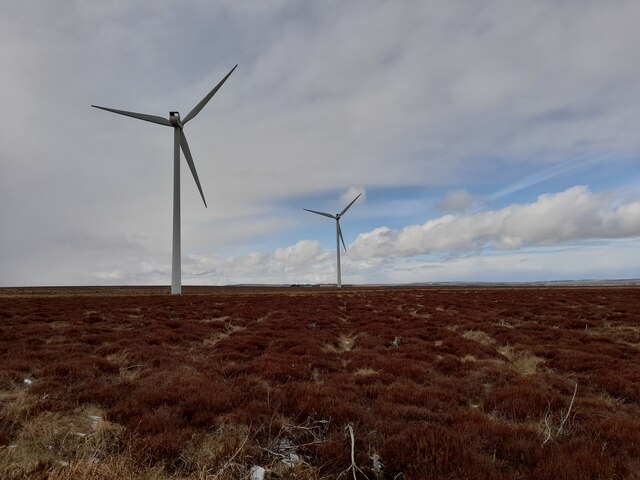In this desolate yet expansive landscape, two towering wind turbines stand prominently against a backdrop of a mostly cloudy sky with patches of blue peeking through. The closer wind turbine is positioned to the left, while the one further back is centered in the photograph. Both turbines are modern, white or gray, and boast three large blades each, designed to generate electric power from the wind. The ground below them is flat and covered with reddish-brown, low-growing plants and brush, interspersed with light-colored grass. The scene evokes a sense of late autumn or winter, indicated by the muted, earthy tones of the vegetation, which includes what appear to be dead flowers or greenery and even some tumbleweed. In the distance, faint hints of buildings and possibly hills or mountains can be discerned, though the area is mostly uninhabited, providing an ideal setup for harnessing wind energy. The field also contains scattered bits of what looks like white trash, adding a touch of stark realism to the scene.